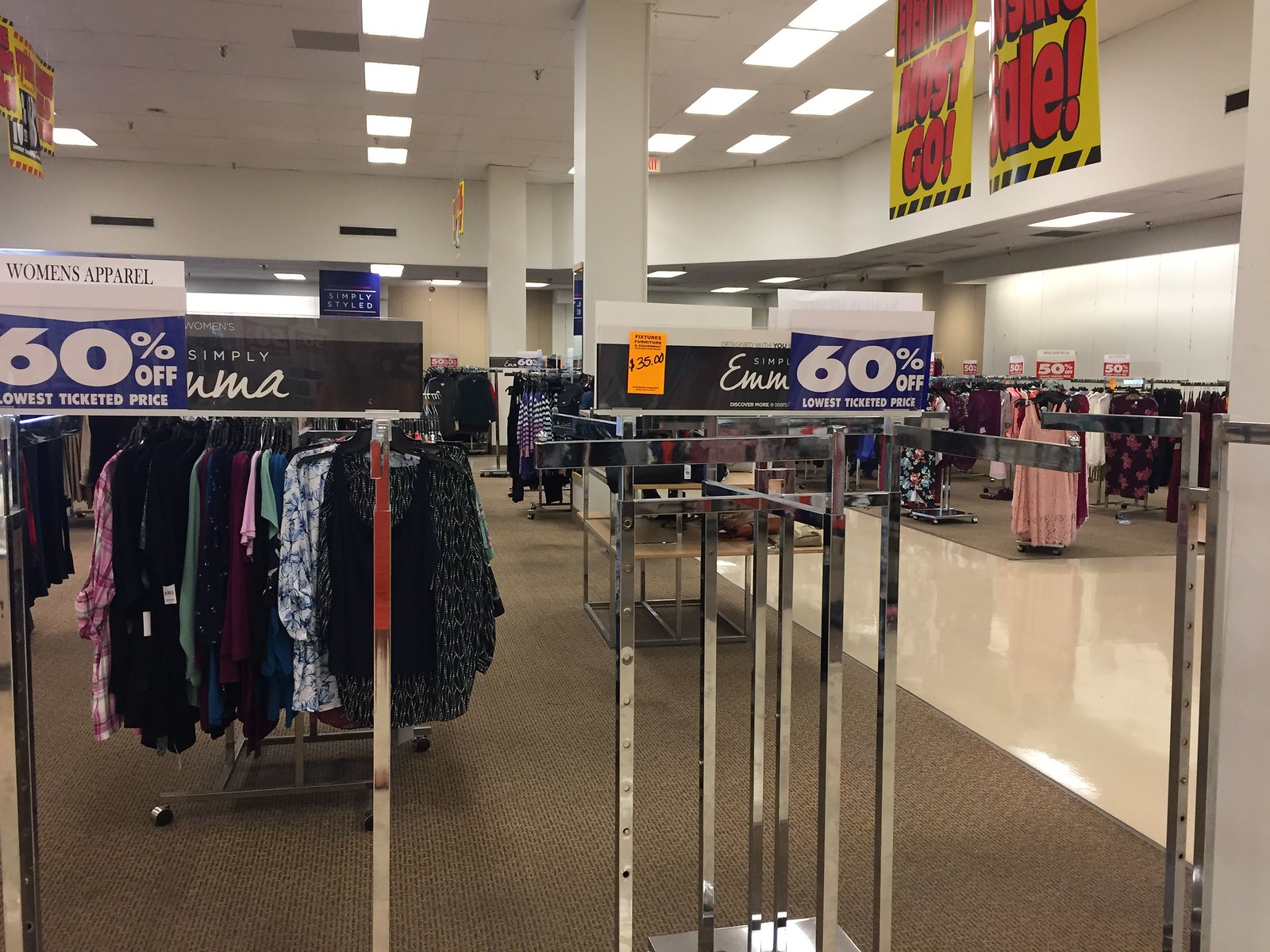The image depicts a first-person view inside a discount clothing retailer, likely a department store, featuring a combination of highly polished white linoleum walkways and commercial gray carpeted areas under the chrome clothing racks. The high ceiling is fitted with drop ceiling panels and recessed fluorescent lights. Two prominent yellow banners with red lettering in the top right corner announce a 'must go' sale. The women's apparel section is highlighted, with a sign on the left indicating 'Women's Apparel 60% off, lowest ticketed price', positioned in front of two empty steel racks. Nearby, a rack is filled with blouses and tops, marked by black rectangles with 'Simply Emma' in cursive. The store layout lacks specific aisles, instead using freestanding racks, with white, bare walls providing a stark contrast to the colorful sale signs and polished floors.